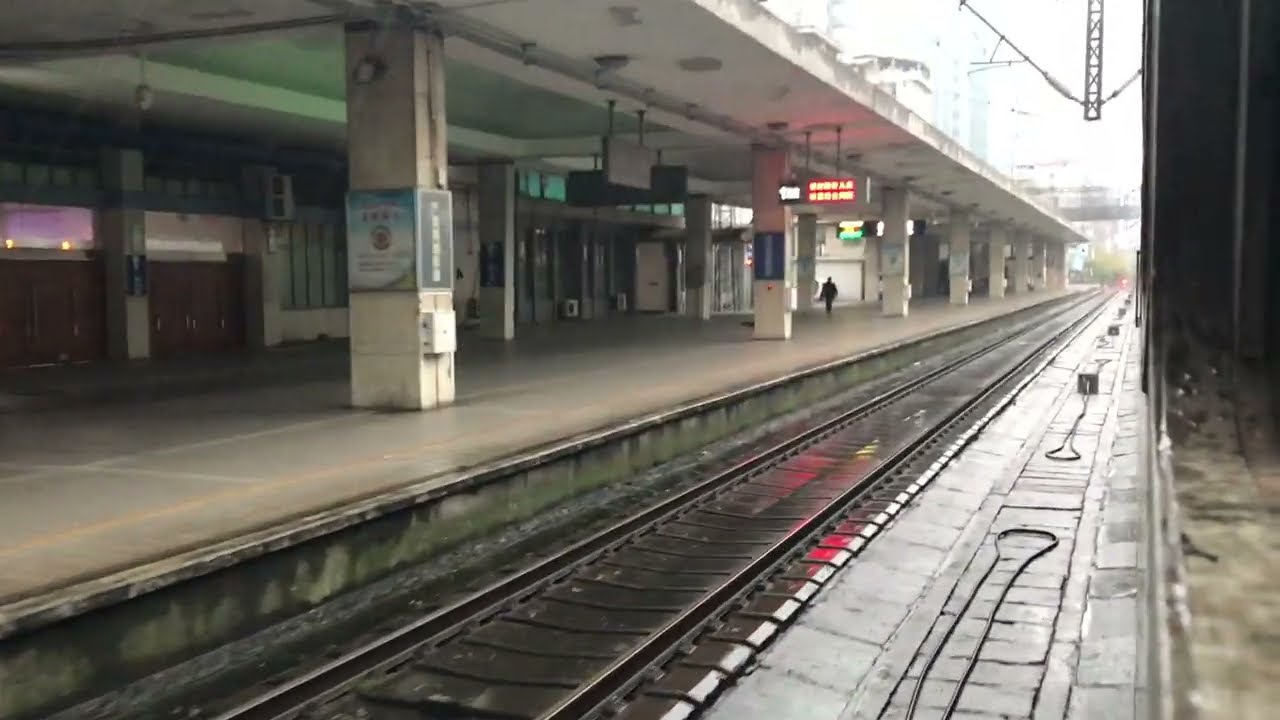The image captures an outdoor train station with a platform to the left, featuring square, white, and somewhat worn-out columns supporting a roof. The platform, which is empty save for one person walking in the center-right of the image, extends under a structure with visible doors and windows. The sky above is bright and overcast, casting a gray, subdued light over the scene. The train tracks, located in the center and right of the image, appear wet, suggesting recent or ongoing rain, although the covered area of the station remains dry. The overall mood is bleak and desolate, with no signs of activity or additional people around. A red sign is visible in the center of the image, though its text is indiscernible, reinforcing the quiet, somber atmosphere. The photo seems to have been taken from the perspective of someone inside a train, with a hint of a window pane visible on the right edge, as they look out onto the empty, rain-soaked station.